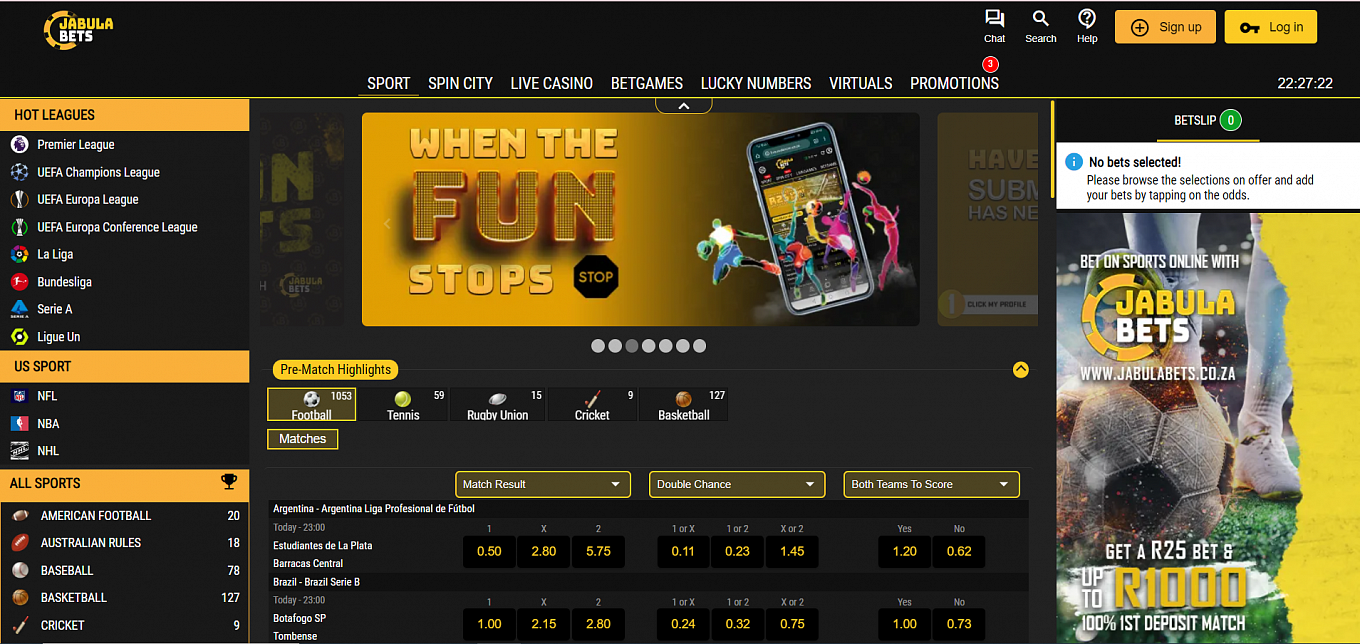This screenshot displays a gamer's website set against a sleek black background. In the upper left corner, a distinct logo catches the eye—a three-quarters orange circle interspersed with the name "JABULA" in bright yellow and "BETS" in bold white text. Stretching across the black header is a menu written in white text, listing options from left to right: SPORT, SPIN CITY, LIVE CASINO, BET GAMES, LUCKY NUMBERS, VIRTUALS, and PROMOTION. The upper right corner features two conspicuous yellow action buttons, labeled SIGN UP and LOG IN, the latter accompanied by a tiny black key icon.

On the left side of the page is a navigation bar topped with a section labeled HOT LEAGUES, highlighted against a gold background. Below this section, in white text on a black background, are several league options each marked with a small circular icon. These leagues include the PREMIER LEAGUE, UEFA CHAMPIONS LEAGUE, UEFA EUROPA LEAGUE, UEFA EUROPA CONFERENCE LEAGUE, LA LIGA, BUNDESLIGA, SERIE A, and LIGUE 1.

To the right, a bright pop-up stands out against an orange background. In bold yellow text, it warns, "WHEN THE FUN STOPS," positioned next to a black STOP sign icon. Additionally, the pop-up displays a colorful image of a cell phone surrounded by four animated players, each holding a basketball, energetically dancing around the screen.